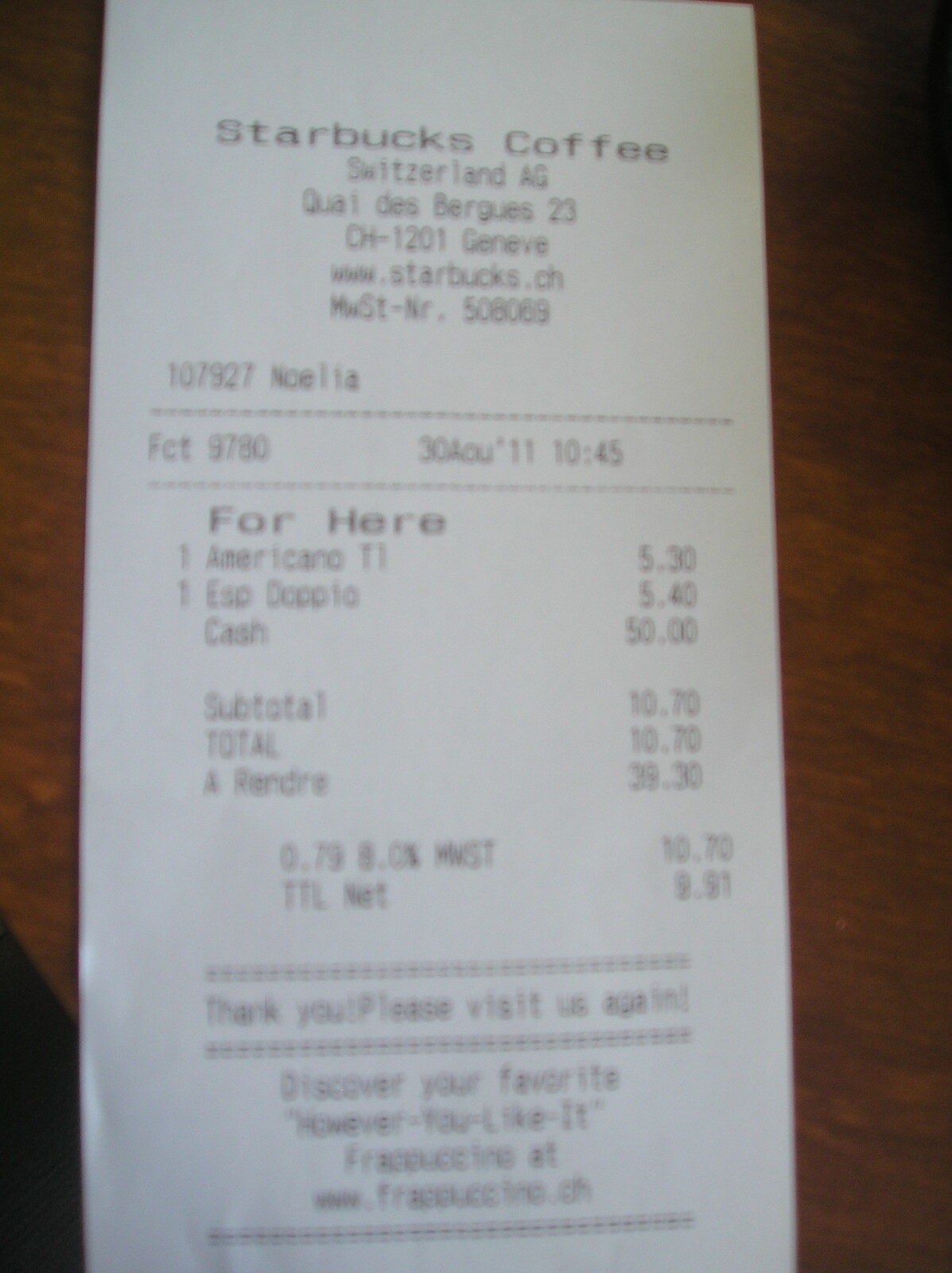An image of a Starbucks receipt from Switzerland, featuring a detailed breakdown of the order placed on August 30, 2011, at 10:45 AM. The receipt bears the name "Noelia" and lists two items: an Americano and an Espresso Doppio. The subtotal for the order is $10.70. Printed at the bottom are the phrases "Thank you, please visit us again" and "Discover your favorite Frappuccino," followed by a blurry website URL. The receipt also includes the order number 107927.